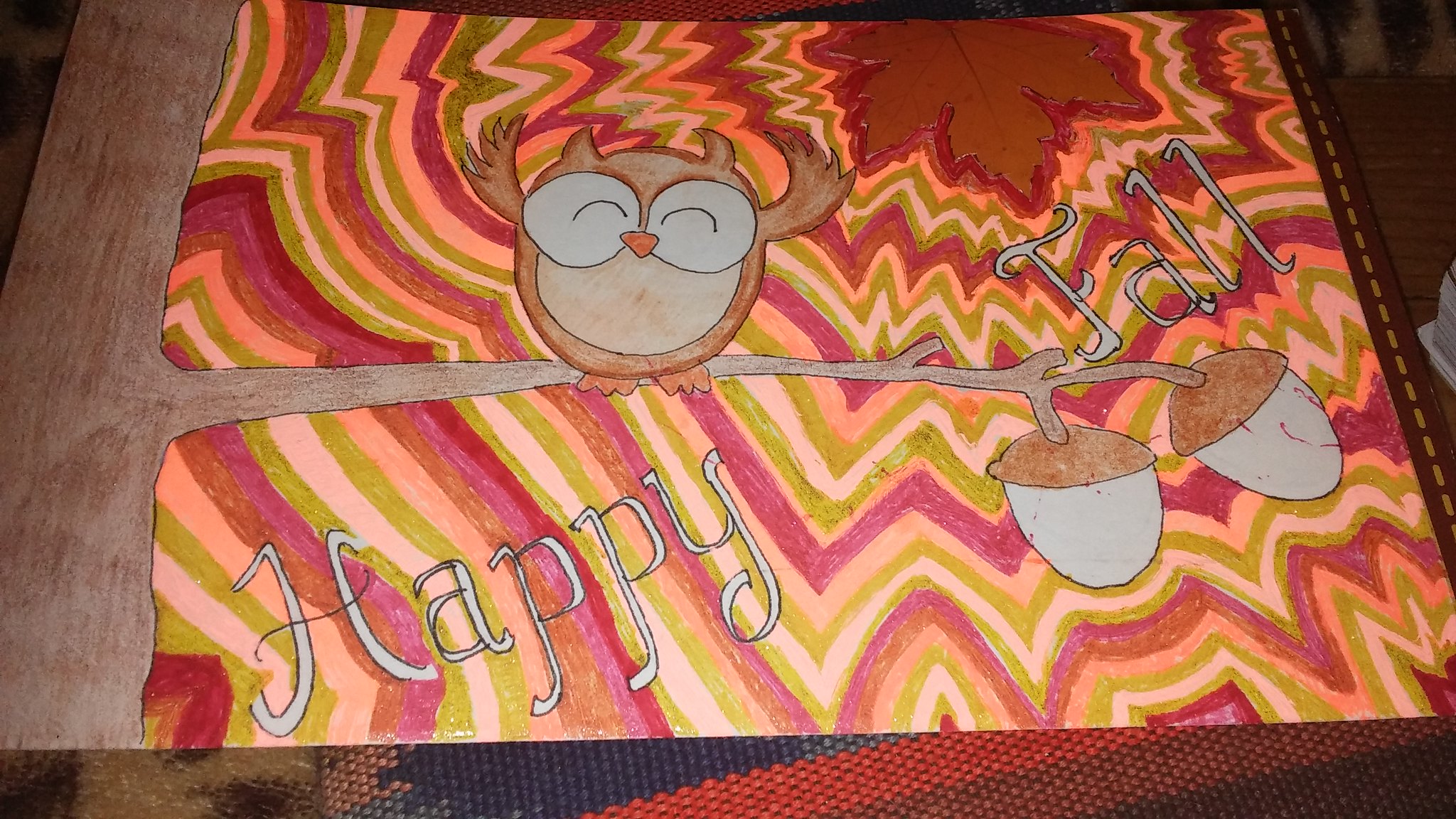The image is a photograph of a detailed drawing on poster board, placed on top of woven striped fabric and possibly a fuzzy animal print blanket. The central figure in the drawing is a cartoon Tootsie Pop owl wearing glasses. The owl, with a dark brown outer body and a tan stomach, has an orange beak and is perched on a tree branch on the left side of the image. The tree trunk is brown and about a third of the way up, the branch extends to the right, holding two acorns with brown tops and white bodies. The owl's wings are raised up, displaying its little feet.

A flowing "Happy Fall" message is displayed across the image, with "happy" written under the branch and "fall" above it on the right. The background features a striking design of angular stripes in colors including lime green, cream, maroon, orange, and peach, radiating from a single point in the top right corner of the drawing, where a large leaf is affixed.